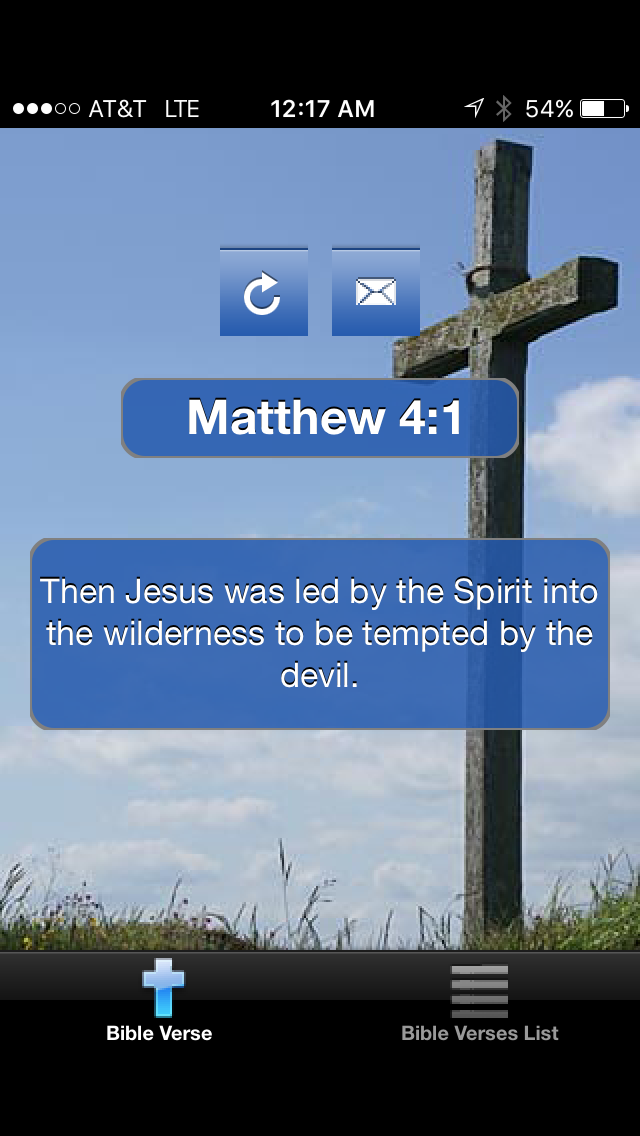This is a detailed description of a screenshot taken from a smartphone, specifically displaying an image with Easter-themed content. At the top of the screen, there's a black border indicating the phone's status, including the service provider "AT&T LTE," the time "12:17 AM," a battery indicator showing "54%," and an envelope icon suggesting unread messages. 

The main image showcases a worn gray wooden cross standing in a grassy field with a few flowers, set against a blue sky. The cross is central in the image with the text "Matthew 4:1" in white letters across a blue bar. Below this, the verse reads, "Then Jesus was led by the Spirit into the wilderness to be tempted by the devil."

Towards the bottom of the image, near the lower left corner, there's a small blue cross icon. Directly underneath this, the text "Bible verse" is displayed in white letters. To the right, five vertical gray lines appear, followed by the text "Bible verses list" in gray letters.

The colors predominantly featured in the image include white, blue, green, and gray, providing a serene and contemplative feel to the Easter-themed display.